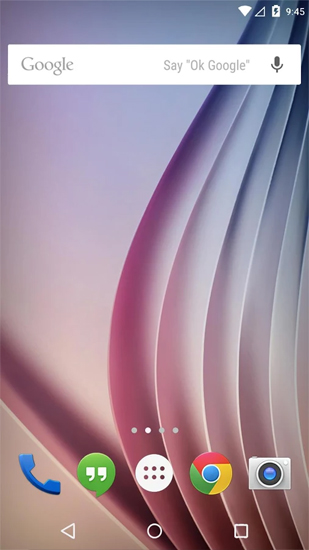This morning, I took a photograph with a background that transitions from pink at the bottom to blue at the top. The time on the device in the image shows 9:45 AM, and the battery icon indicates that it is currently charging, denoted by a thunderbolt symbol. The home screen prominently features the Google Search bar at the top, accompanied by the "Okay Google" phrase and a microphone icon. Below this, there is an array of four dots, with the second dot highlighted in white while the others remain gray.

The screen displays a variety of app icons. Notably, there is a blue phone icon, a green chat icon, a white circular icon containing two rows of three smaller circles that resemble a perforation in a larger circle, the Google Chrome icon, and a camera icon. At the bottom of the screen, there are navigation buttons in the shape of a triangle (left arrow), a circle, and a square, signifying the back, home, and recent apps functions respectively.